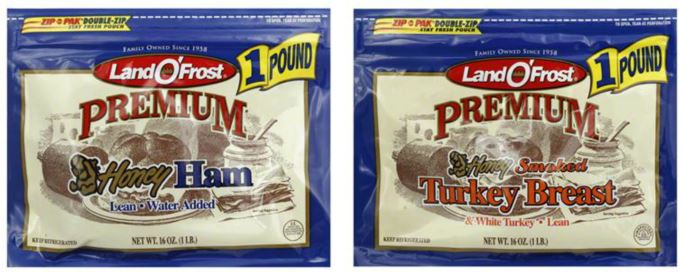This image showcases two rectangular, blue packages of deli meats from the brand Land O’ Frost, each adorned with a white label, red oval brand logo, and yellow accents. The package on the left proudly displays "Premium Honey Ham" in bold letters and features an illustration of ham and honey. The honey ham package, marked with a yellow banner in blue letters, indicates a net weight of 16 ounces, equivalent to one pound. It also highlights its lean quality with added water and a resealable "Ziploc Zip-Pack" top. To the right, an almost identical package features "Honey Smoked Turkey Breast" with the same overall design elements, including the net weight and resealable functionality. Both packages emphasize ease of use with their resealable tops, ensuring freshness for multiple uses.